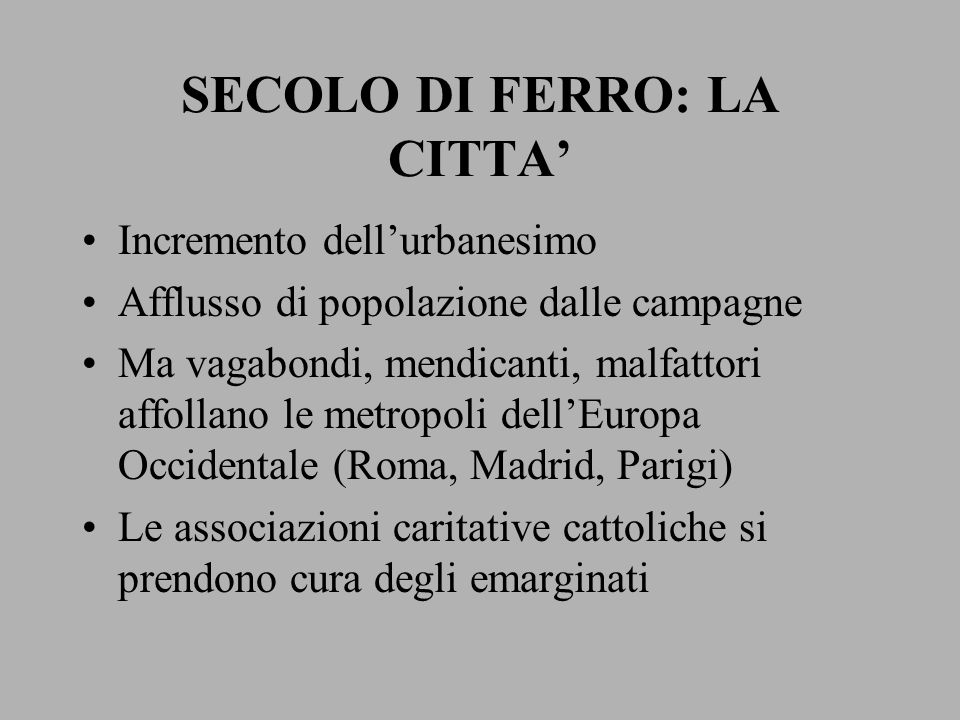The image features a solid light gray square background with black text in Times New Roman font. At the top, centered and in bold capital letters, it reads "SECOLO DI FERRO: LA CITTÀ." Below this title, four bullet points are listed. The first bullet point states "incremento del urbanissimo," indicating an increase in urbanization. The second point, "afflusso di popolazioni dalle campagne," refers to the influx of populations from the countryside. The third bullet point describes a more complex situation: "ma vagabondi, mendicanti, malfattori affollano le metropoli dell'Europa occidentale" (with cities like Rome, Madrid, and Paris specifically mentioned in parentheses). Finally, the fourth bullet point notes the role of charitable Catholic associations: "le associazioni caritative cattoliche si prendono cura degli emarginati," which translates to their efforts in taking care of the marginalized.